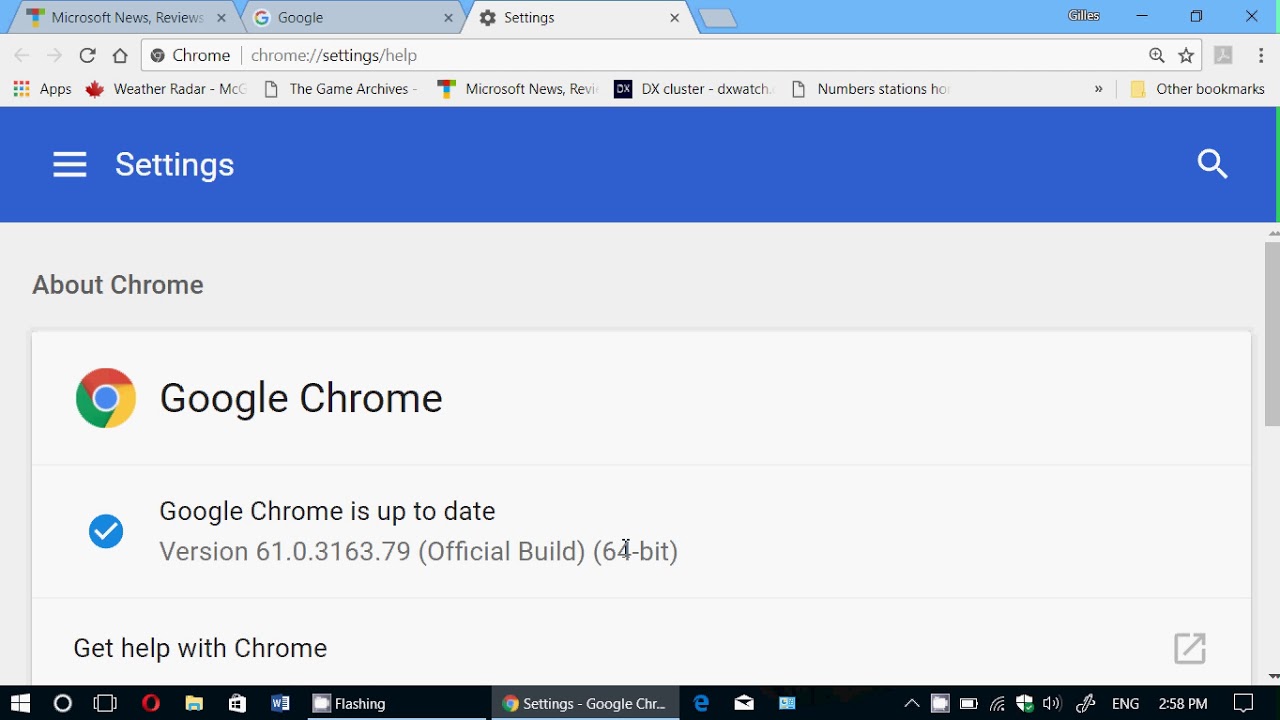The image is a screenshot of the Google Chrome settings page, specifically under the "Help" section. At the top, the URL bar displays "chrome://settings/help." The left sidebar contains a navigation menu with "Settings" prominently listed at the top. On the right side of the page, there is a magnifying glass icon representing the search function. 

Below the settings menu on the left, "About Chrome" is noted, and next to it, the Google Chrome icon is displayed. Just below, a blue circle with a white check mark indicates that "Google Chrome is up to date." The version information is listed as "Version 61.0.3163.79" followed by "(Official Build)" and "(64-bit)" in parentheses. At the bottom of the sidebar is an option that reads, "Get help with Chrome."